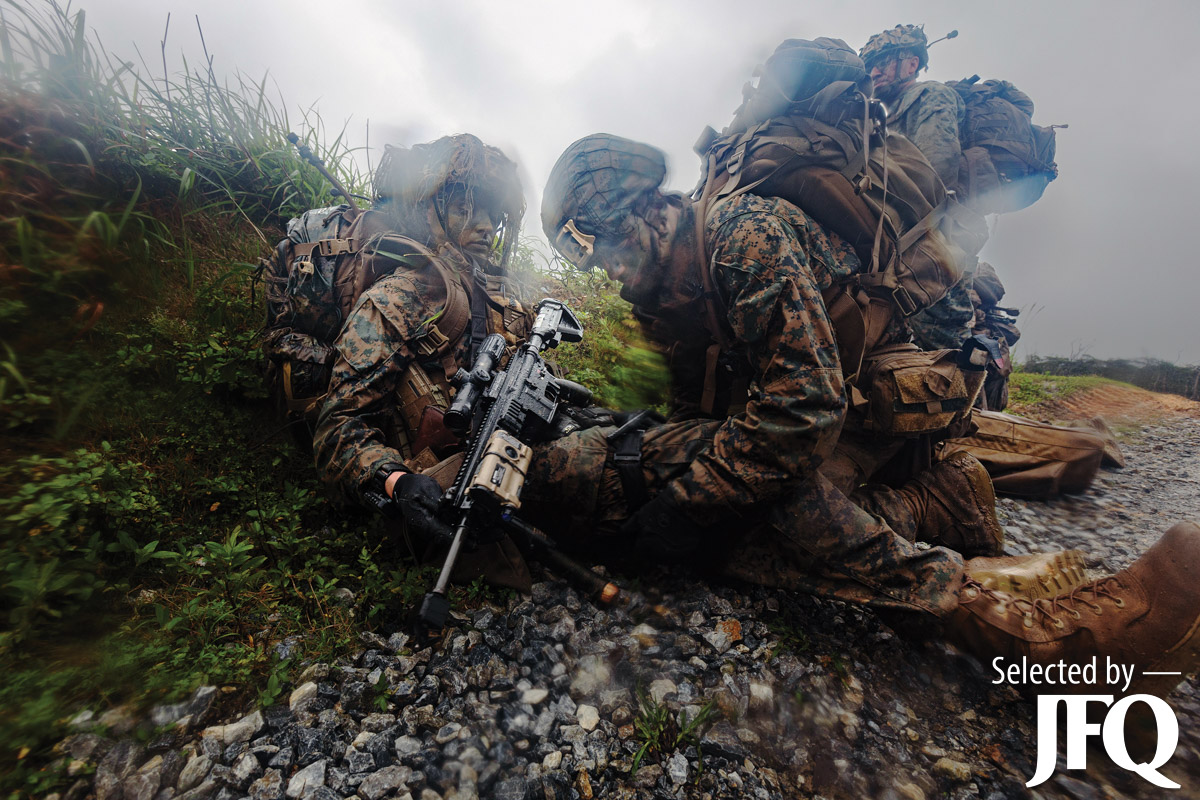In this detailed image, three U.S. soldiers are captured in an intense battlefield moment, likely set in Afghanistan. The soldiers are fully geared in camouflage uniforms and helmets, with face paint for additional concealment. The picture focuses closely on them as they seem to seek cover beside a small bush on a gravelly terrain. The two soldiers in the foreground are seated as if fatigued or possibly injured. One soldier has his rifle resting against his body and looks exhausted, while the other seated soldier appears to be slightly leaning back, his left arm reaching around the first soldier's leg, suggesting either a gesture of support or tactical maneuvering. Both have rucksacks on their backs.

In the background, a third soldier stands, possibly overseeing the situation or providing assistance. This soldier is equipped with a large rifle and wears radio equipment along with glasses, indicating a communication role. An overcast sky dominates the backdrop, suggesting a recent rainfall, adding a somber, wet ambiance to the scene.

In the bottom right corner of the image, white text reads "SELECTED BY JFQ," with "JFQ" in bold capital letters, providing a stark contrast to the earthy tones of brown, green, grey, and blue that dominate the picture. The overall mood conveys a powerful mix of tension, exhaustion, and determination amidst the rigors of war.